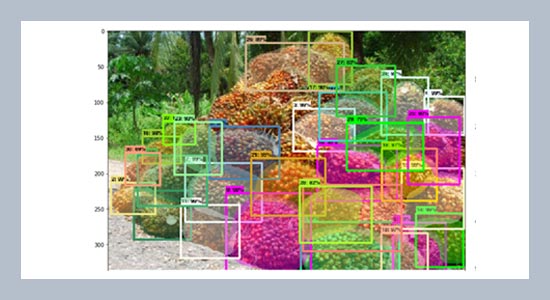The image is a small rectangular photograph with a gray border and white matting. It features a colorful depiction of a flower garden set on a mound, abundant with hues of pink, green, and orange flowering plants. The garden scene also includes a few boulders atop the mound and is bordered by green forested woods in the background. A gray gravel pathway is visible at the bottom left corner, running along the edge of the flower mound. 

Overlaying the photograph are numerous neon-colored rectangles in shades of green, yellow, white, beige, orange, and purple. These rectangles overlap each other, each framing sections of the garden in various combinations of colors. Accompanying each box are notations too small to read, likely detailing the contents within each framed area. To the left side of the image, a vertical scale numbered from 0 at the top to 300 at the bottom suggests a graph-like element. The photograph maintains a style of photographic realism combined with graphic design elements.